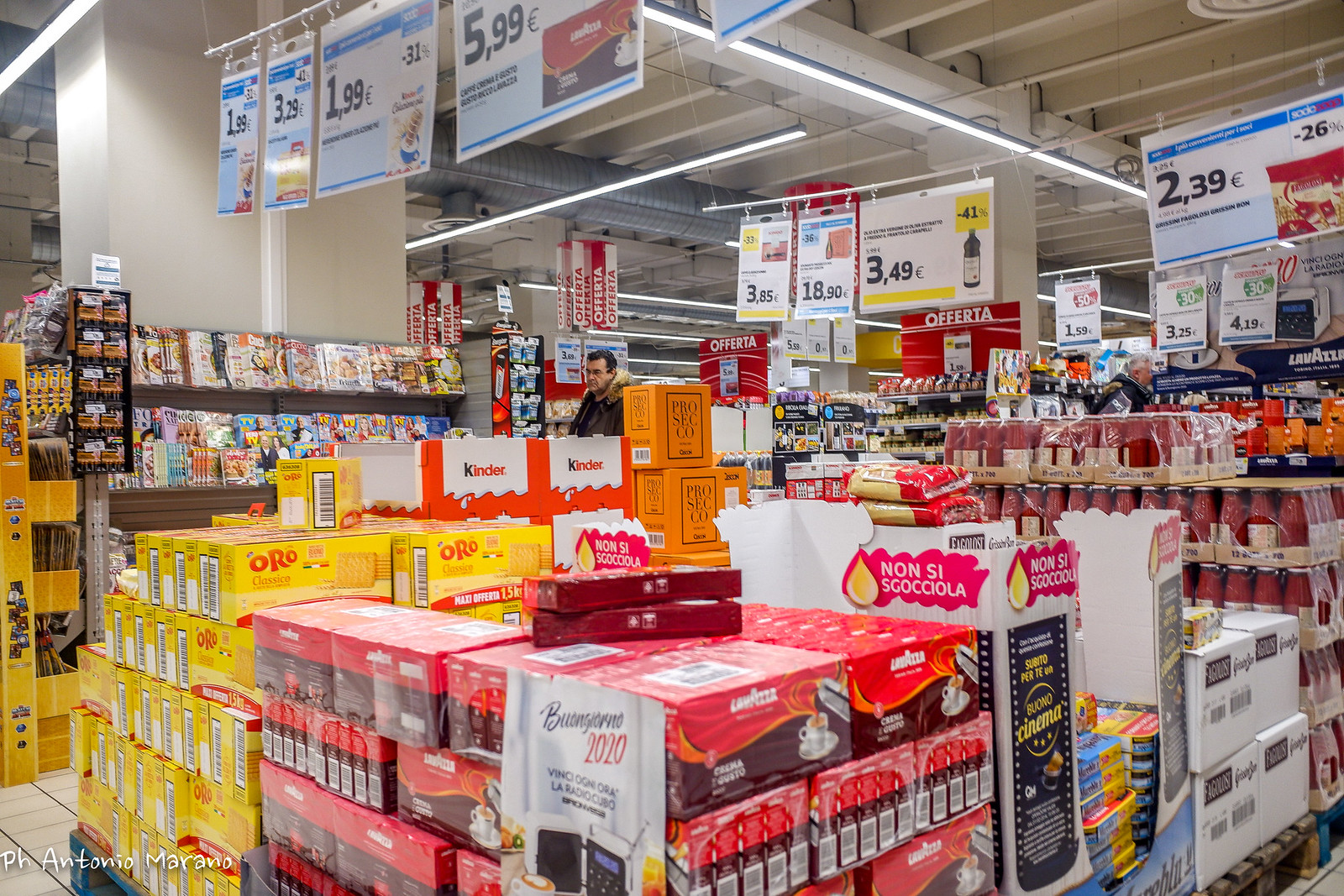The image depicts the interior of a bustling market, which appears to be a combination of a grocery and department store. The scene is rich with various items and large discount signs or promotional banners in Spanish or Italian, all priced in euros. Centered in the foreground, several pallets on the ground are stacked with bulk goods, including Lavazza coffee, Oro Classico biscuits, Kinder eggs, and what seems to be ketchup. These products are encased in red and brown packaging. A prominent book and magazine shelf is visible to the left, with racks of magazines at eye level. In the bottom left corner, white text reads "PHANTONIO MARANO." The store is lively, with two men present in the background, contributing to the scene's dynamic atmosphere. The store's consistent red and white branding on signage further adds to the visual coherence of the setting.